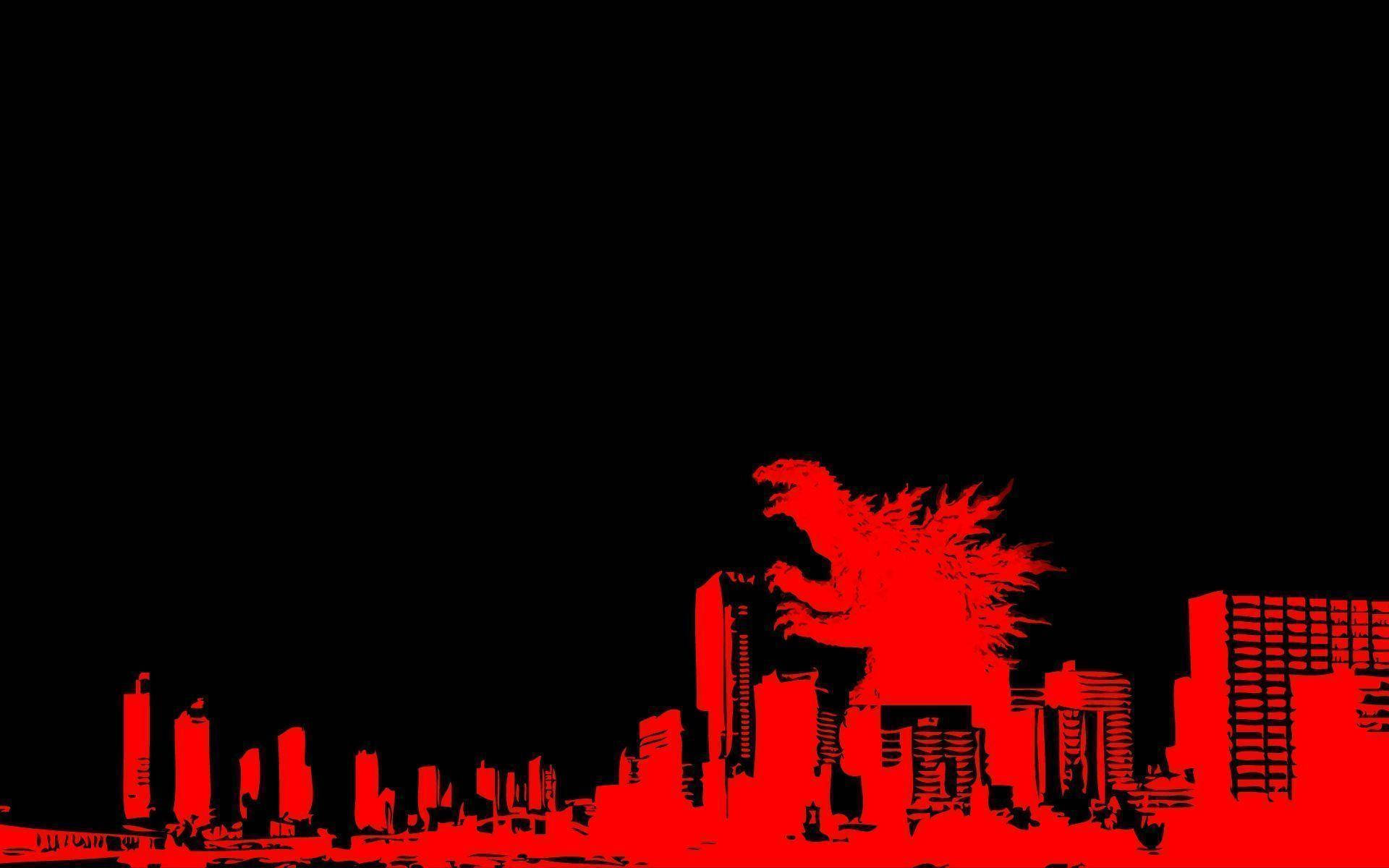This illustration is a computer-rendered, cartoon-style depiction of Godzilla attacking a city, presented in a rectangular landscape format. It features a striking palette of red and black. The entire backdrop of the image is a solid black, representing a night sky without any additional details. The action is concentrated in the bottom half of the image, where a cityscape of varied skyscrapers is depicted in vivid red hues. This cityscape includes a variety of building types, from wide and tall to thin and tall, and stretches to the left with some buildings partially obscured. The tallest skyscraper, situated at the center, reaches about two-thirds the height of Godzilla.

Godzilla, also rendered entirely in red, dominates the scene. Positioned behind the buildings in the right center, the creature is depicted standing and facing to the left. It walks on two legs with its front limbs extended, appearing ready to attack. The spikes on its back resemble flames or wild brambles, contributing to its menacing appearance. Godzilla’s mouth is open as if growling, adding to the intense atmosphere of the scene. In the foreground on the right, a large apartment building can be seen, further grounding Godzilla's immense size in relation to its surroundings. A bridge crossing an implied body of water is faintly visible, adding depth to the urban landscape.